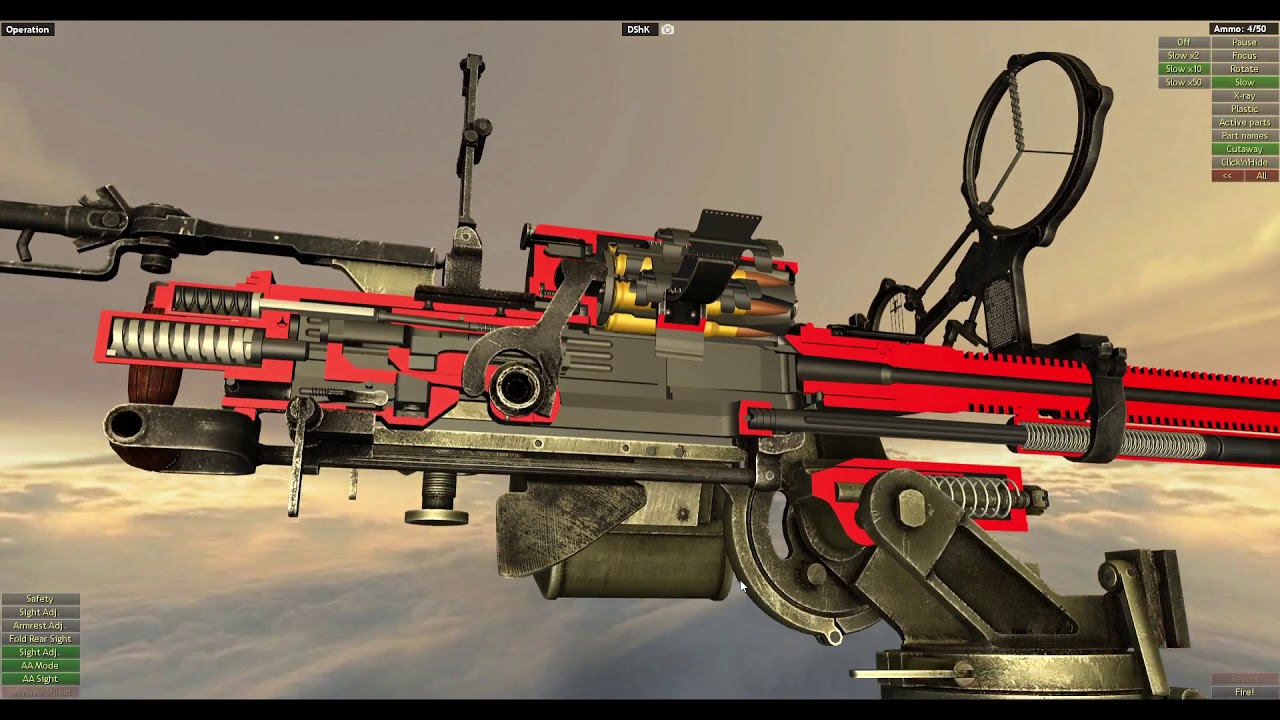The image is a detailed close-up of a large turret or gun, likely from a video game, possibly Call of Duty. The turret is positioned prominently in the center, with the barrel extending towards the middle-right. The gun is adorned with various attachments and mechanisms, creating a busy appearance. Notable features include a black scope at the back and long, gold bullets with brown tips. The gun's colors are predominantly red, black, and silver, with other elements accented in dark green and orange-ish hues, resembling bullet casings. The background sets the scene high in the sky amidst gray clouds with hints of yellow and beige, suggesting a sunrise or sunset. Subtle detailing reflects advanced graphics, showcasing scuffed, brushed, or polished hardware. Text appears in the top right and bottom left corners, though it is too small and blurry to read clearly.